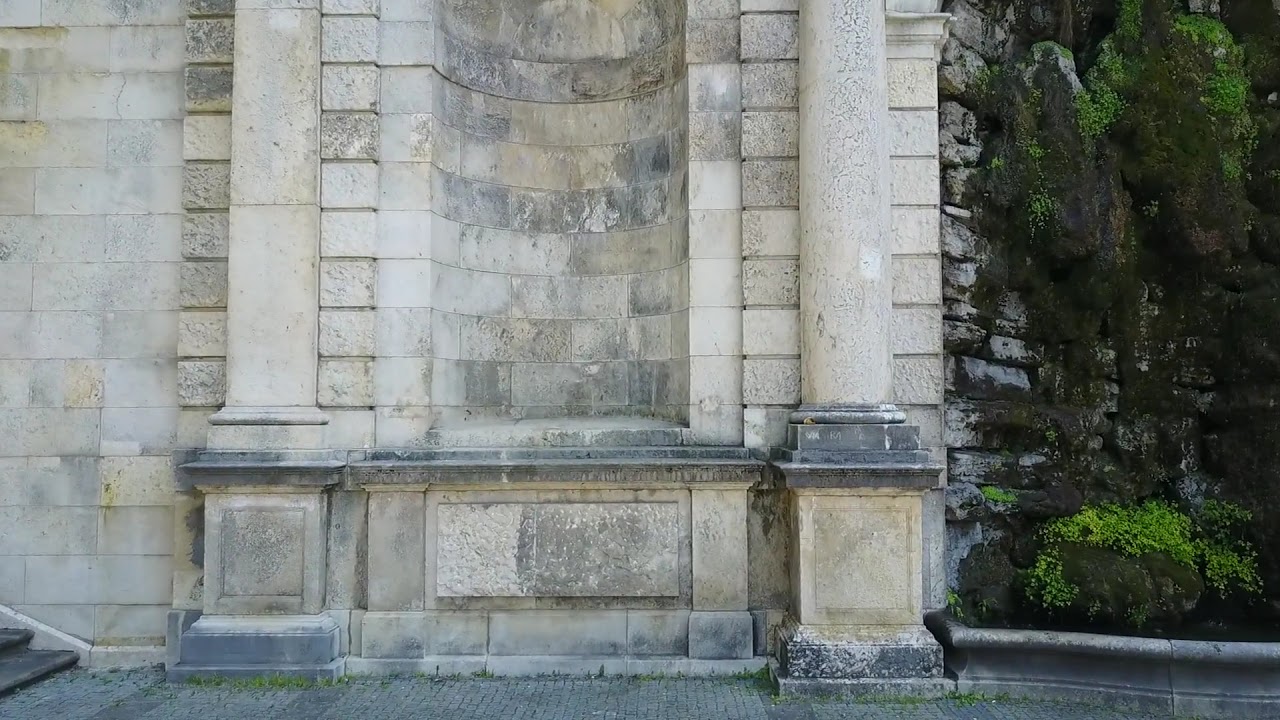The image depicts the side of a large, vintage stone building with a light beige or cream-colored facade. Dominating the middle and left two-thirds of the horizontally oriented photograph are two prominent cream-colored columns, each resting on concrete bases positioned in front of a natural stone wall. The columns seem to frame a recessed area decorated with ornate stonework, perhaps once hosting a statue. Below this architectural detail is a gray stone path or sidewalk. To the left of the image, in the bottom left corner, there are partial views of stairs that appear to lead off-frame. The right third of the image transitions to a rugged, green moss-colored rock wall with a concrete edge at the bottom, accompanied by some green foliage near the lower part. The setting is outdoors during the daytime, with ample natural light illuminating the scene, devoid of any human presence.